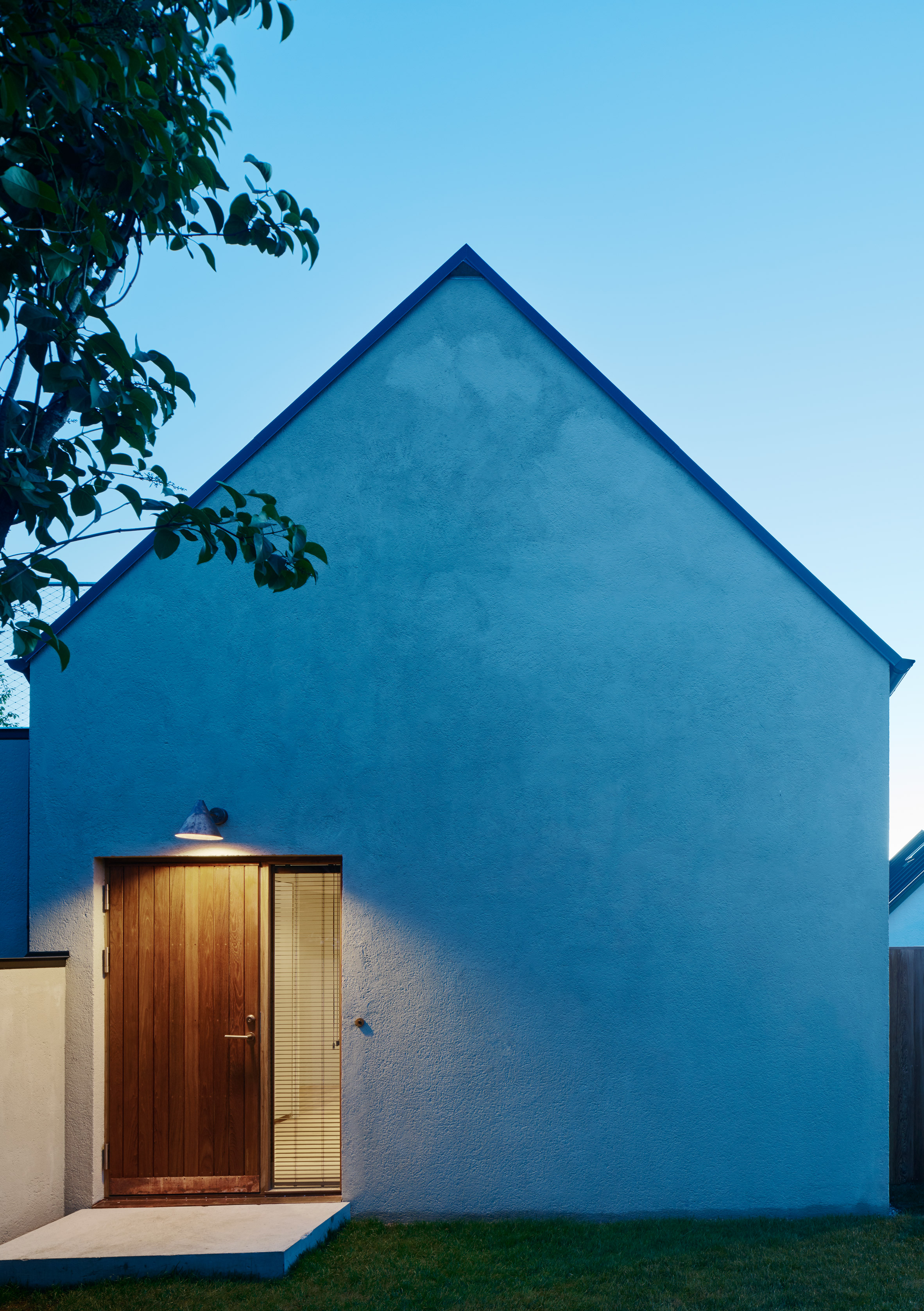This photograph captures a minimalist white stucco house under a twilight blue sky, where gradient hues transition from light to dark. A steel, triangular blue roof tops the structure, adding a sharp, geometric contrast to the smooth walls. The front face of the house is strikingly plain, devoid of windows, except for a prominent door on the bottom left. This door, crafted from vertical wooden planks with a rich brown finish, is framed by black hinges, a metal handle, and a keyhole. A narrow, long window with partially opened mini blinds accompanies the door, hinting at a warmly lit room inside. Above, a farmhouse-style conical spotlight shines down, casting soft light on the concrete entryway. The surrounding atmosphere includes short green grass and a single tree with overhanging branches on the left. To the right, a faint glimpse of another fence and roof suggests neighboring structures. The composition indicates an early morning or evening setting, lending the scene a serene, almost timeless quality.